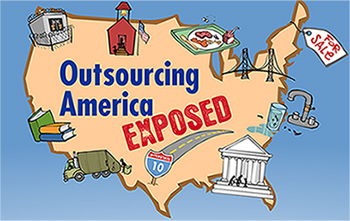This illustration features a blue background with a pink outline of the United States at the center. Dominating the image are the words "Outsourcing America" in blue, with the red, slanted word "Exposed" underneath. Various icons are dispersed across the map. In the upper-left corner, over Oregon, there is a building with a barbed wire fence resembling a prison compound. To the right of that, a stack of three books in green, yellow, and blue is placed where California would be. Over New York, an iconic bridge is depicted. In the Midwest, particularly over Minnesota, there's a tray of food. The lower section of the map shows a garbage truck near Arizona, and a road along with an Interstate 10 sign. The right side of the map, particularly over the eastern states, includes a spigot, symbolizing water, and a "For Sale" tag tied to Maine. Over Florida, there is a white government building with columns indicating a congressional building.